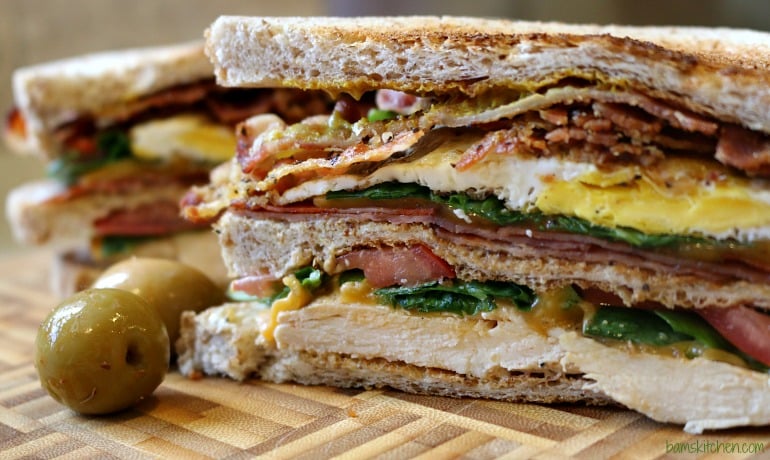In this photo, we see two beautifully assembled half sandwiches, each meticulously crafted with three layers of toasted white bread. The top layer of the sandwich features crispy bacon, a perfectly fried egg with a bright yellow yolk and white part, along with fresh greens. The middle layer is comprised of a slice of bread followed by juicy tomato slices, more greens, and succulent slices of chicken. The entire creation is topped off with another slice of toasted bread. This detailed cross-section reveals the richness and variety within each sandwich.

Adjacent to the front sandwich, two green olives are delicately placed. The sandwiches rest on what appears to be a bamboo placemat, with the background featuring a similar, albeit blurred, sandwich setup. The sandwiches are noted for their appealingly toasted flatbread, arranged in tow on a clean, grey surface. Despite the elegance and careful construction, there is no text directly within the photo itself. However, a watermark on the bottom left corner reads "bam bam's kitchen.com". Overall, the image is a feast for the eyes, suggesting a delightful and hearty combination of flavors and textures perfect for a breakfast or brunch setting.